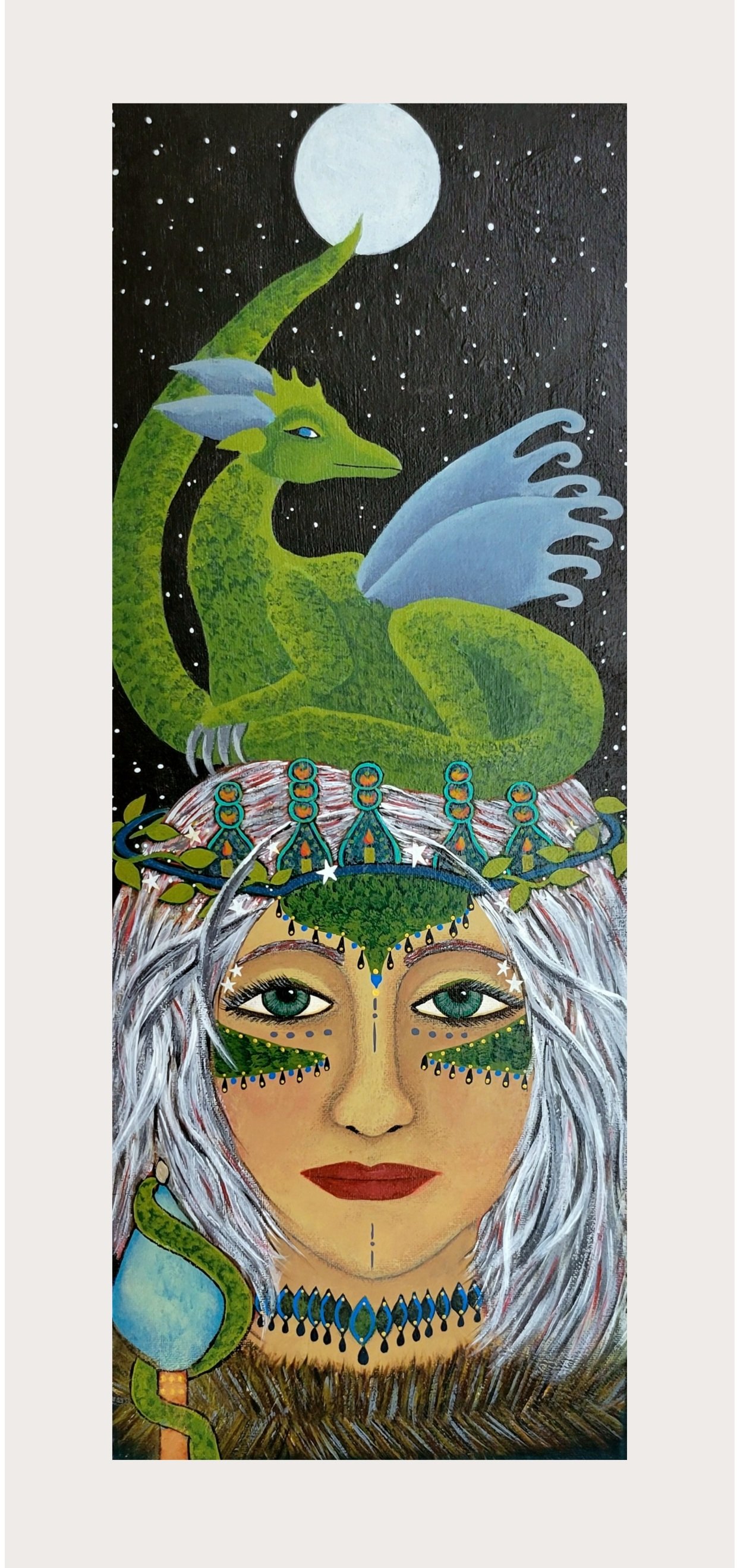A tall, skinny painting with a thick white border all around features a mystical scene in a detailed color illustration. At the bottom of the image is a woman with shoulder-length icy blue-white hair, adorned with green makeup on her forehead and under her blue eyes, and red lips. She wears a headdress resembling a green-scaled crown and a blue necklace with blue triangular pendants. Her attire includes a brown fur collar, and she holds a staff with a blue, teardrop-shaped tip entwined by a green, scaly design. Sitting atop her head is a green dragon with blue wings, ears, and eyes. The dragon is curled up, its tail extending upward to touch a full moon centered at the top of the image. The background features a black night sky dotted with stars, enhancing the fantasy element of the painting.